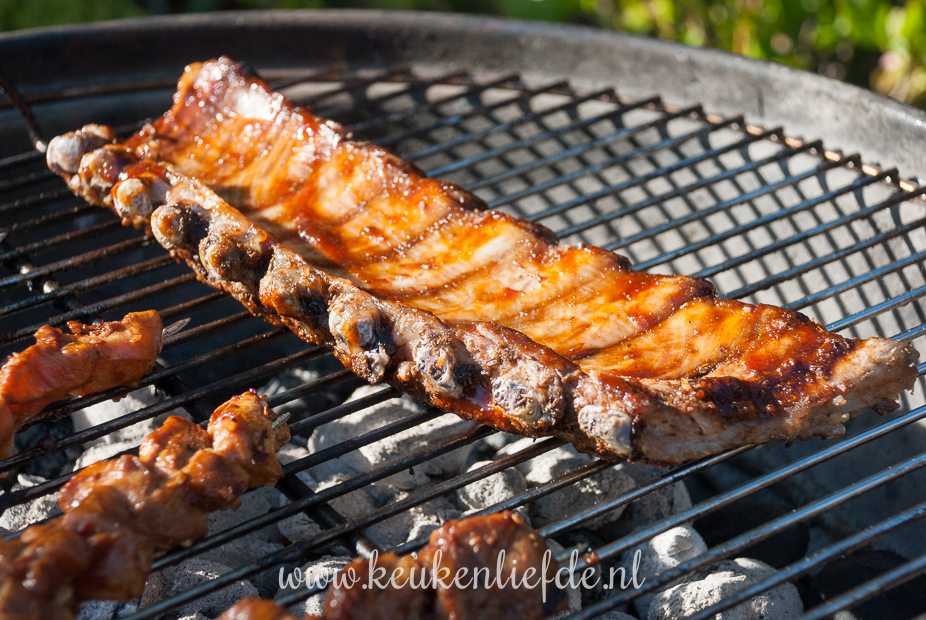A close-up image captures a gray-silver charcoal grill, with glowing white charcoal briquettes underneath. Centered diagonally on the grill rack are ribs coated in an orangish barbecue sauce, showing a mix of reddish, brown, and black colors from thorough cooking. To the side, there are three half-visible kebabs on metal skewers, also coated in sauce, displaying a mix of red, white, and yellow hues. The grill rack is the main focus, with black wires crisscrossing underneath the meat and faint green vegetation blurring into the background. At the bottom of the image, the website "www.keukenliefde.nl" is written in cursive white letters.